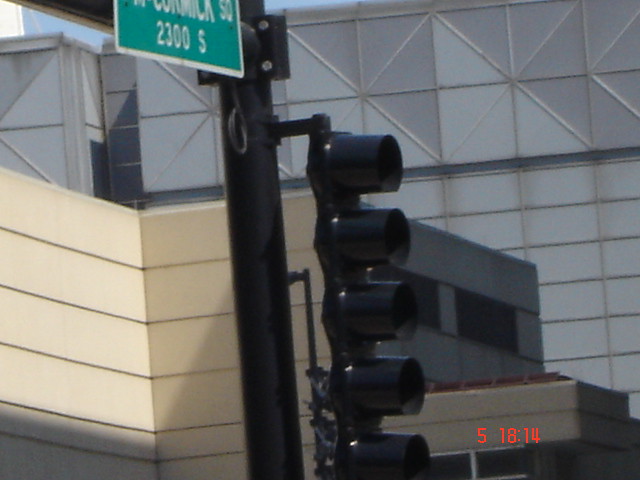This photograph, taken outdoors, primarily captures a black traffic light pole featuring five stacked lights, each surrounded by black frames, facing towards the right. The image is somewhat out of focus and of modest quality. A timestamp in red, reading 5 18 14, is visible in the lower right corner, indicating the photo was taken at 6:14 PM. Above the traffic light, a partially cut-off green street sign displays "2300 S" and an unclear street name, likely "Cormula." In the background, a modern white building with a distinctive geometric pattern of diamond shapes at the top and rectangular shapes at the bottom is visible. Additionally, the bottom left corner of the image shows an off-white wall.